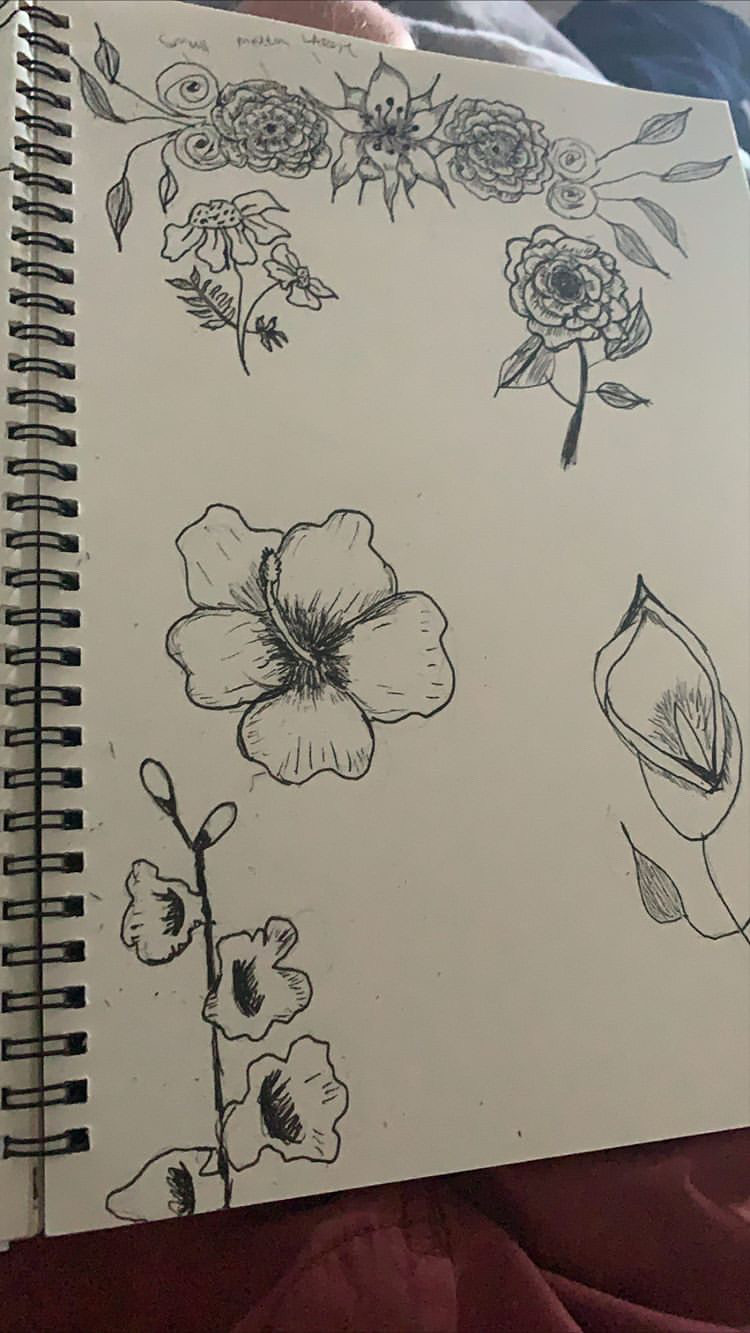This photograph showcases an open spiral-bound sketchbook lying on a crumpled reddish bed comforter. The black metal spirals on the left-hand side hold the pages in place. At the top of the visible page, a delicate banner formed by different flowers and leaves stretches across the width. Below the banner, the page features intricately detailed black ink sketches of various flowers, including a daisy, a rose, two types of orchids, a lily, a hibiscus, a hydrangea, and some daisies and bluebells. Also visible in the image are parts of the artist's leg at the top and their pants at the bottom, adding a personal touch to this creative scene.